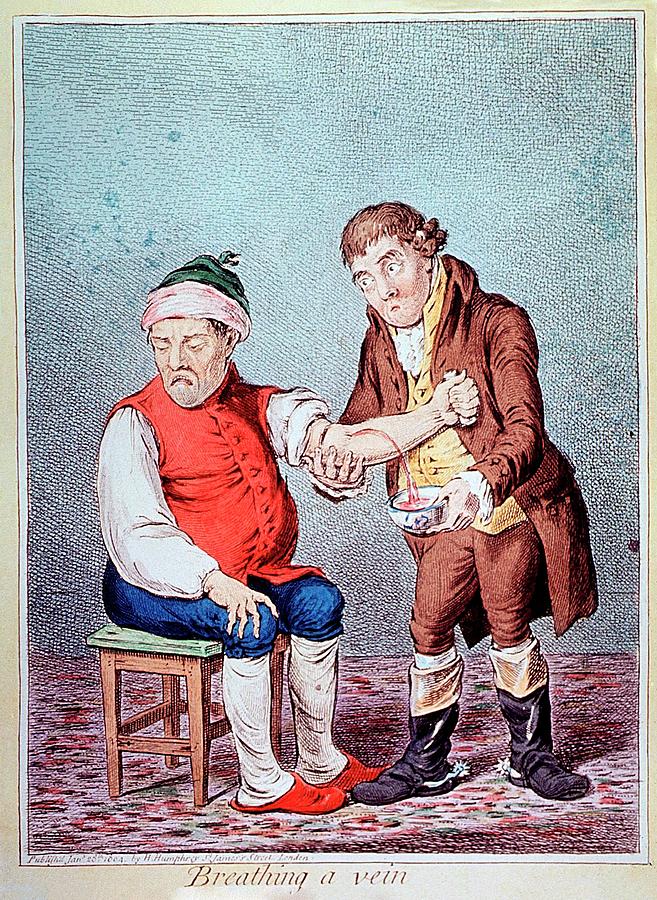This image, titled *Breathing a Vein*, is an older, colored drawing that depicts the historical medical practice of bloodletting. The scene features two short and stout characters, rendered in what appears to be a late 1800s art style. The central figure on the left, the patient, wears a bright red vest with puffy white sleeves, blue pants, and long white socks that reach his knees, along with red slipper-like shoes. He also has a distinctive headwrap or hat with a white brim and a green top with a tie. Sitting on a small footstool, the patient looks away, gripping an object to tense his arm as blood arcs from a single puncture into a bowl held by the doctor.

The doctor, in period-appropriate attire, wears a brown waistcoat, yellow button-up shirt paired with what appears to be a white cravat, and matching brown pants. His brown hair features curls on the sides, and his footwear includes boots with a golden fold at the top and spurs. Despite the lack of conventional medical instruments, the doctor simply holds the patient’s arm to perform the procedure. They are set against the backdrop of a blue wall and an ornate, though low-resolution, pink carpet with red and green patterns.